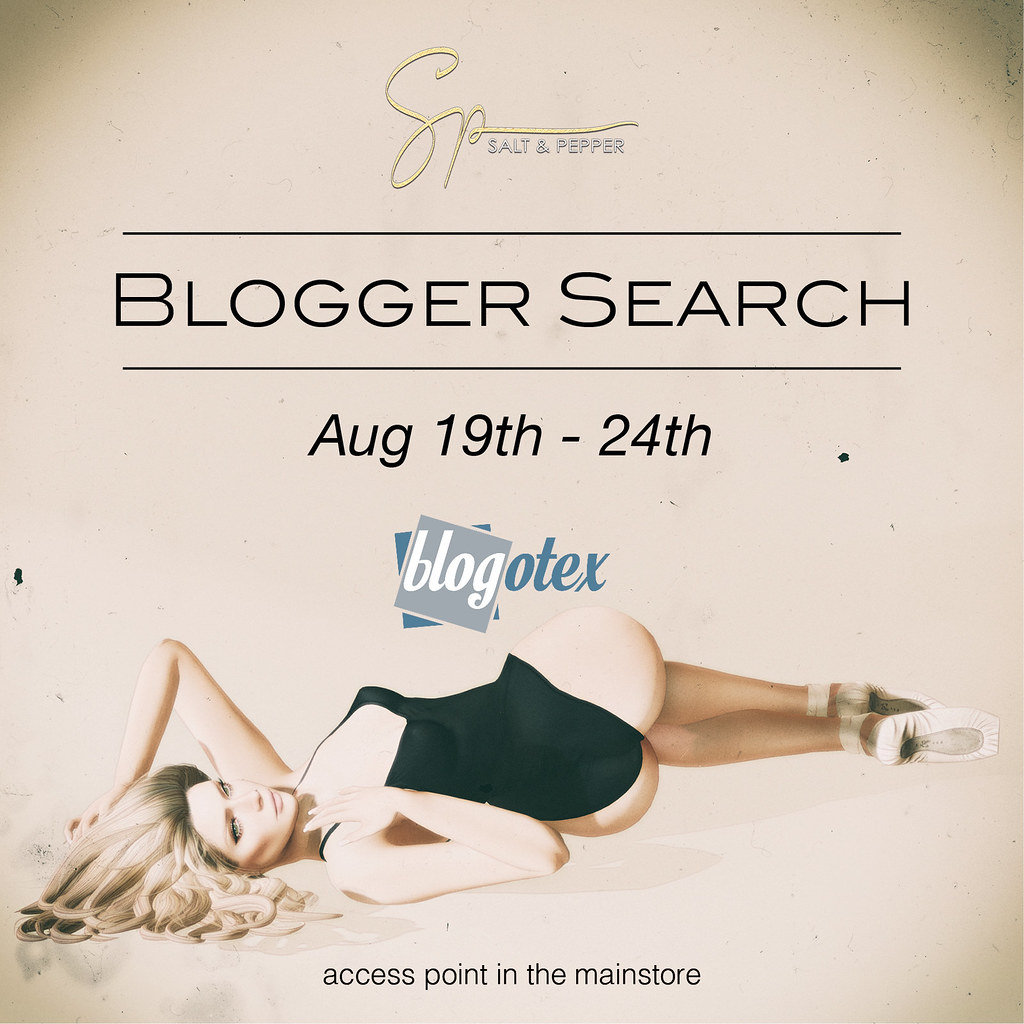The image is a square-shaped poster with a light pink background. At the top middle, there's a yellow logo that reads "SP" with the word "Salt and Paper" in white. The logo features an extended line under the "P" that underscores "Salt and Paper." Just below the logo, in large capital letters, is the phrase "BLOGGER SEARCH," flanked by black horizontal lines above and below. The dates "AUG 19th to 24th" are written in italicized text beneath this. Below the dates, the word "BLOGOTEX" appears. Dominating the lower portion of the poster is a detailed illustration of a blonde woman wearing a black one-piece ballet-like outfit and white ballet flats. Her hair is splayed around her head, and she is posed lying back with her arms folded. Directly beneath her illustration, in lowercase letters, is the text "access point in the main store."